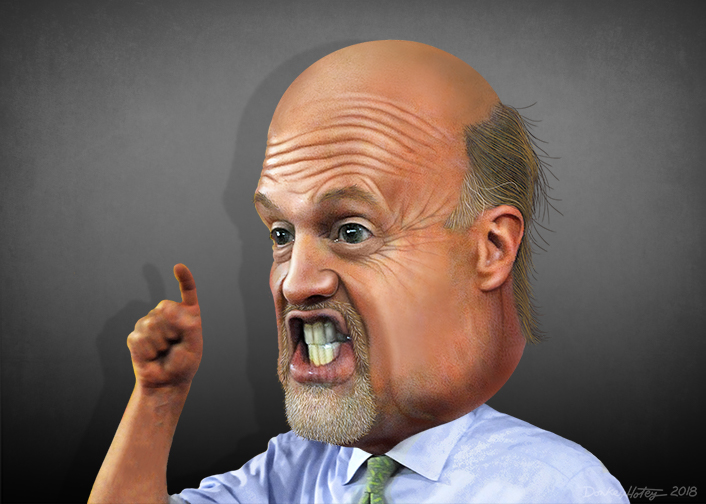The image is a detailed caricature, capturing stock market analyst and economic forecaster Jim Cramer. The illustration features an exaggerated depiction of his head, which is notably larger than his smaller, attached shoulders. His head is bald on top with some gray hair on the sides, and he has a distinctive short beard, goatee, and a bit of a mustache. His facial expression includes tightly together teeth and lips, with visible wrinkles around his eyes and forehead, enhancing his characteristic features. He has squinty eyes and pronounced jowls, adding to the caricature's vividness.

Cramer is depicted wearing his signature light blue button-up shirt with rolled-up sleeves and a patterned green, somewhat beige tie. His right arm is bent at the elbow, with his finger prominently pointed upwards, emphasizing a point he seems to be making. His mouth is open slightly, showcasing his teeth. The caricature is set against a light and dark gray background with a vertical rectangular layout. The name "HOTEY" is signed at the bottom left corner, dated 2018.